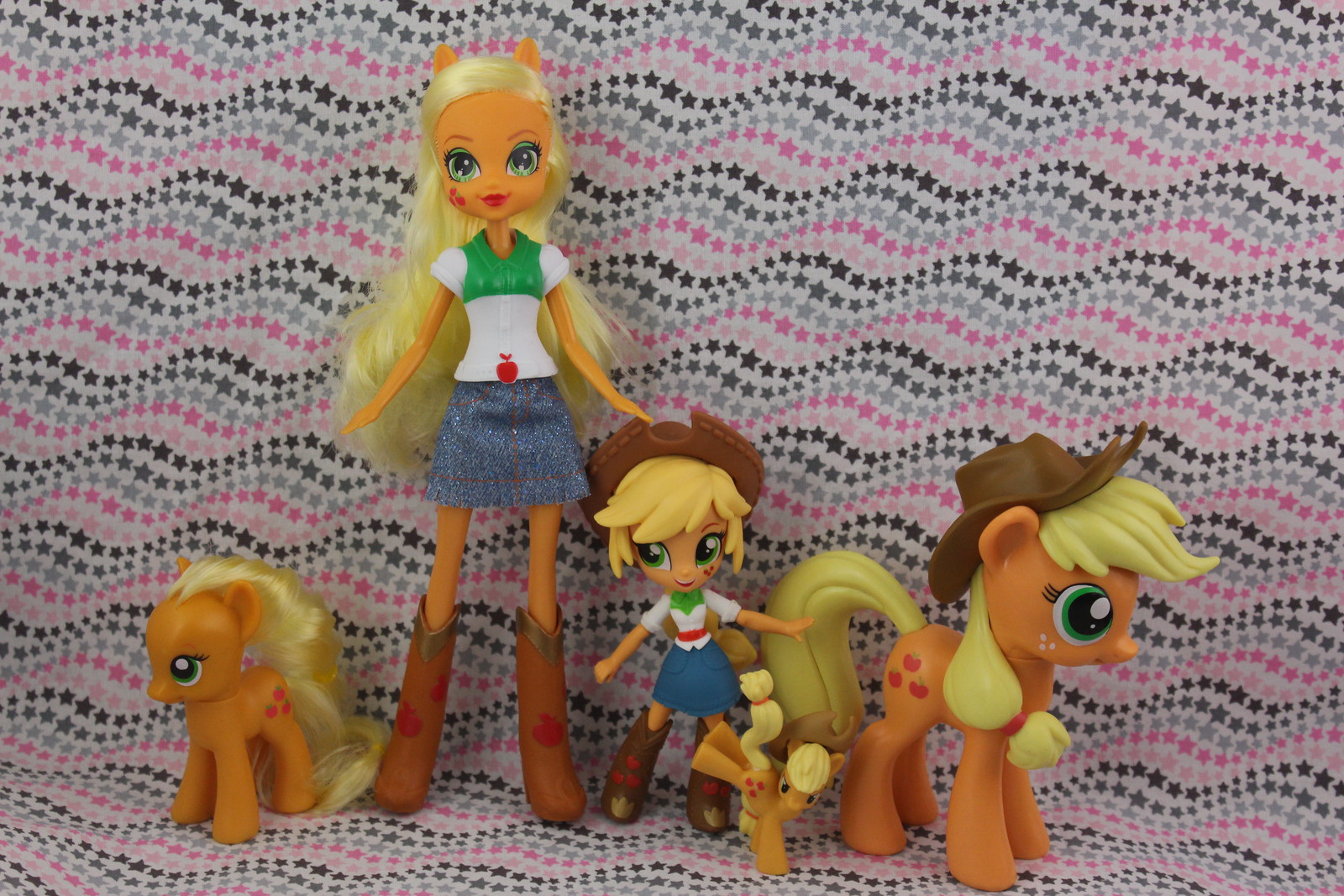The image depicts a chaotic but vibrant scene with a backdrop of wavy lines of small stars in various shades of pink, gray, and black. At the forefront, two orange My Little Pony figures are positioned facing opposite directions. The pony on the left features yellow hair, while the slightly larger pony on the right sports a brown cowboy hat and has three apple symbols on its flank. Between these ponies stands an adult-sized doll with blonde hair, blue eyes, and a white long-sleeve shirt, accented with green around the chest. She wears a blue denim skirt, a red belt, and brown cowboy boots adorned with three hearts. Additionally, she has a belt buckle in the shape of an apple. To her right is a shorter plastic female figurine, similarly dressed in cowboy attire: a white shirt, blue denim skirt, red belt, brown cowboy boots, and a brown cowboy hat, mirroring the taller doll's appearance. The composition of toys against the starry backdrop creates an engaging and detailed visual narrative.